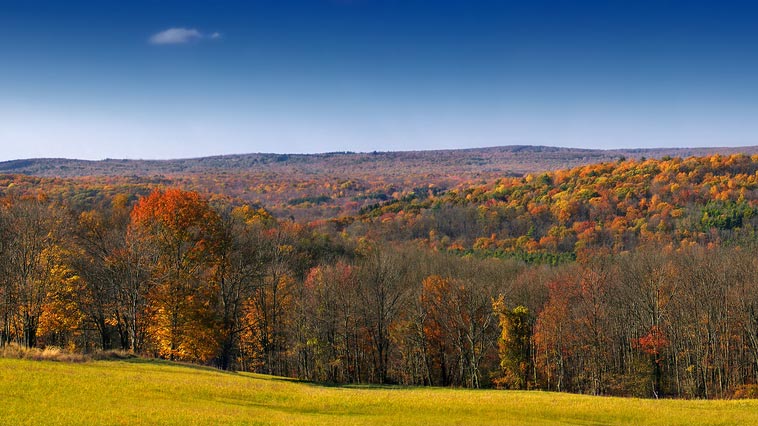This horizontally aligned rectangular image captures a serene, autumnal landscape. Dominating the upper portion is a clear, vibrant blue sky with a singular, feathery gray cloud lingering in the upper left corner. Below, the eye is drawn to a sprawling expanse of mixed foliage that stretches across the majority of the scene. The foreground features short, yellowish-green grass transitioning into myriad trees showcasing the vibrant spectrum of fall—orange, red, yellow, green, and even purples. Among the trees, some branches stand bare, while others are densely adorned with colorful leaves. These trees, with their thin branches and trunks, are interspersed across rolling hills, hinting at the possibility of the area being part of a golf course. The flat land in the distance accentuates the layers of trees vividly changing color in the middle ground, creating a picturesque and crisp autumnal vista.